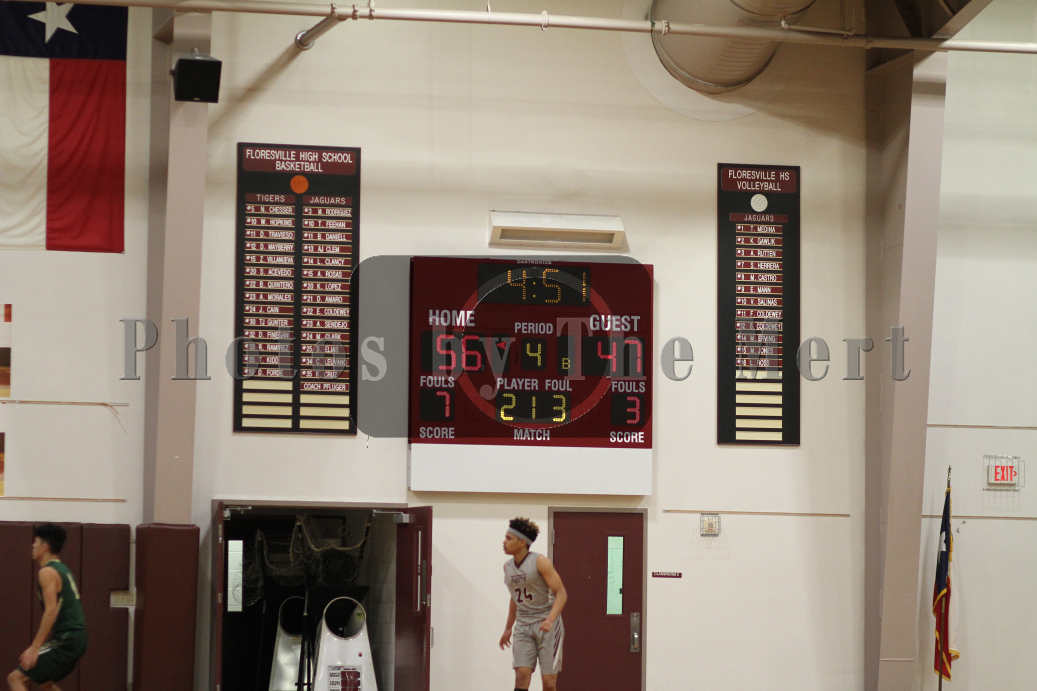This image captures a moment in a high school gymnasium, which is identified as Floresville High School, home of the Tigers and Jaguars. The gymnasium's white walls are adorned with digital scoreboards and various award listings, highlighting the school's achievements in basketball and volleyball. One prominent feature is a digital scoreboard centered on the wall, displaying a game time of 4:51 remaining in the fourth period, with the home team leading 56 to 47. The scoreboard also indicates foul counts and player numbers involved in fouls.

The gymnasium is detailed with red padded areas around beams and posts for safety, Texas and other flags, and black speakers suspended from the ceiling. A pair of red doors at the bottom center, with one slightly ajar, frames the background. 

In the foreground, a player from the home team stands near the doorway. He is partially turned, showing the left side of his face, characterized by an afro secured with a gray headband. Dressed in a gray sleeveless uniform with the number 24 and matching shorts, he contrasts with another player in green visible in the background. A watermark reading "Photos by the MERT" is faintly superimposed across the middle of the image.